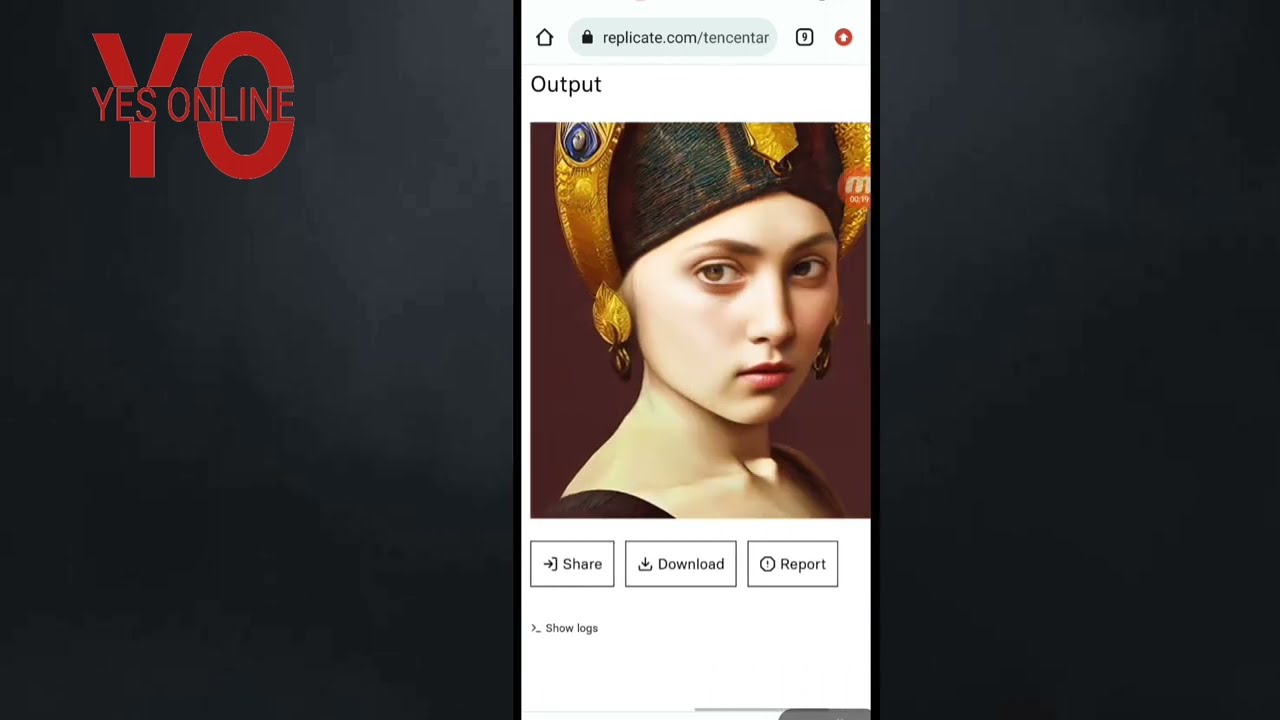The image is a detailed screenshot of a webpage predominantly set against a black-gray background. In the upper left corner, red text spells "YES ONLINE" over the letters "Y-O". Central to the image is a smartphone browser displaying a webpage from "replicate.com/tencentaur", with the browser showing nine open tabs. The page title is "Output".

Within the webpage, there's an image resembling an oil painting of a young girl with a sideways gaze. She is wearing an elaborate headdress that is black with red accents and features a yellow centerpiece, complemented by yellow feather earrings. Her upper attire and background within the painting are also red. The webpage features three interactive buttons: "Share", "Download", and "Report", followed by an option to "Show Logs". The girl's portrait stands out against a white section of the page, contrasting with the primary dark theme of the screenshot. This appears to be an AI-generated image showcased on the "YES ONLINE" template.